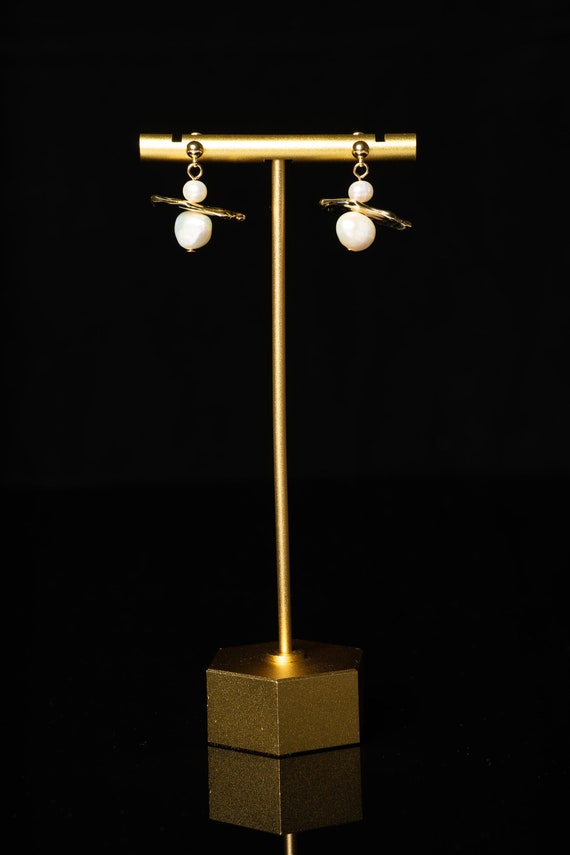The image displays a golden tool, set against a stark black background, with a reflection visible at the bottom. The tool features an octagonal base, from which a vertical pole extends upwards. Perpendicular to this pole is another horizontal pole, forming a T-shape. Hanging symmetrically from each end of this T-shaped rod are ornate golden earrings. Each earring is adorned with a small white pearl at the top, followed by a golden bar and a larger white pearl beneath it, mirroring the design on both sides. The scene is simple yet elegant, with the gold and white elements standing out strikingly against the dark backdrop.